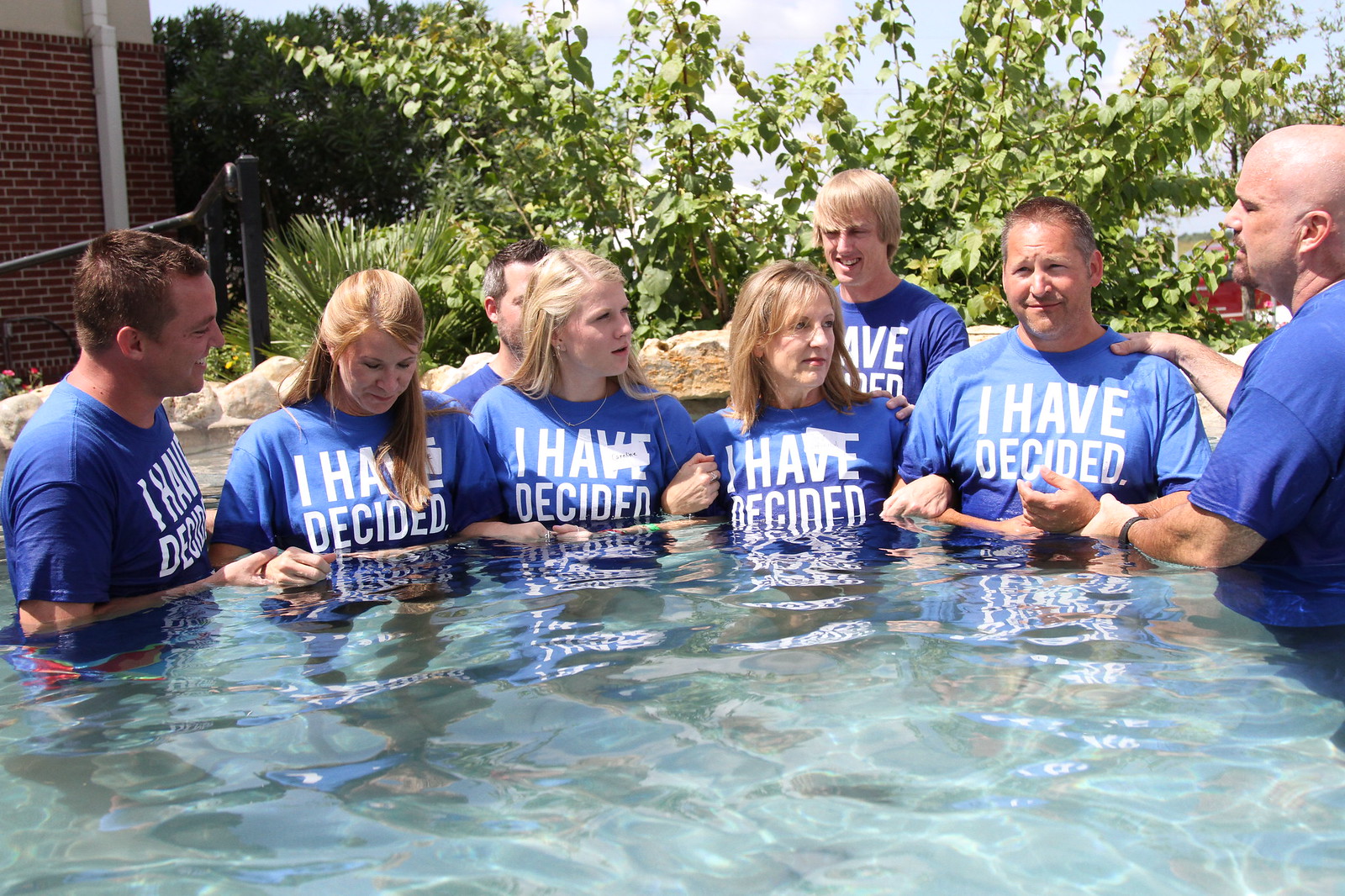In this photo, a group of eight people, all dressed in blue shirts emblazoned with the phrase "I Have Decided," stands together in a swimming pool. The group comprises individuals who appear to be related, with the two people on the right side likely a mother and father, and the younger individuals possibly their children, based on their appearance. Notably, the man on the far right has a bald or shaved head and a goatee, and he places one hand on the father's shoulder while his other hand rests on the father's wrist. 

The individuals in the photo are predominantly white, with most of them having blonde or light brown hair. Their arms are interlocked, suggesting unity and support among the group. Surrounding the pool is a faux rocky ledge, enhancing the naturalistic setting, and a bush is visible in the background. 

The overall atmosphere appears to be one of happiness and solidarity, though the context of their gathering is not immediately clear. The caption suggests a possible ritualistic element, possibly connected to the declaration on their shirts. Despite the unknown specifics, the group's expressions of contentment hint at a positive and meaningful shared experience.